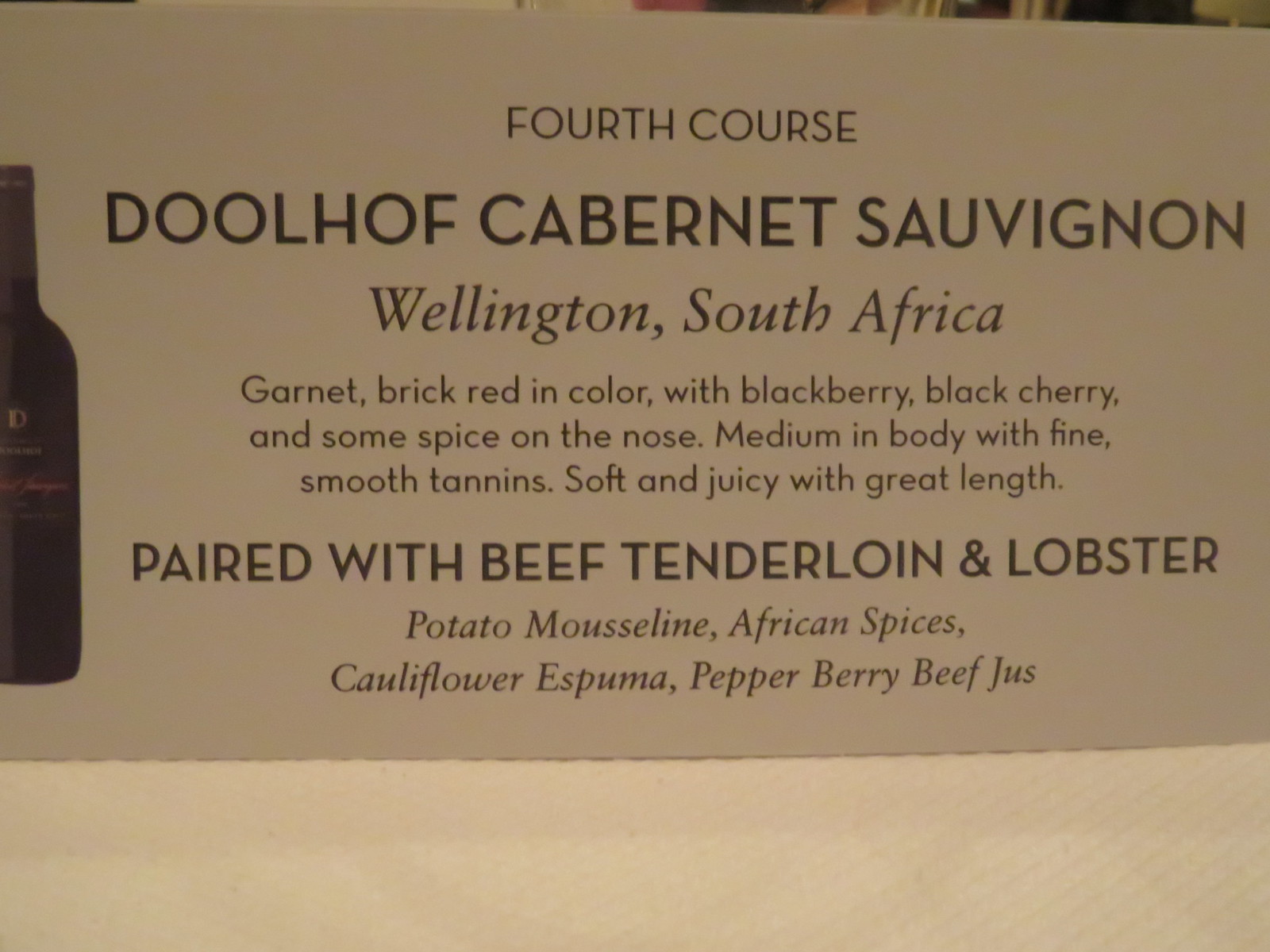The image is a photograph of a menu card primarily featuring the fourth course of a meal. At the top, in bold text, it reads "Fourth Course," followed by "Doolhof Cabernet Sauvignon, Wellington, South Africa." The wine is described in detail as "Garnet, brick red in color with blackberry, black cherry, and some spice on the nose. Medium in body with fine, smooth tannins, soft and juicy with great length." Below this, in larger text, it states that the wine is "paired with beef tenderloin and lobster." The accompanying dish includes "potato mousseline, African spices, cauliflower espuma, and pepper berry beef jus." On the left side of the text, there is an icon of a wine bottle, though it is partially cut off in the image. The overall card appears to be in black and white with minimal color and is simply printed on paper.